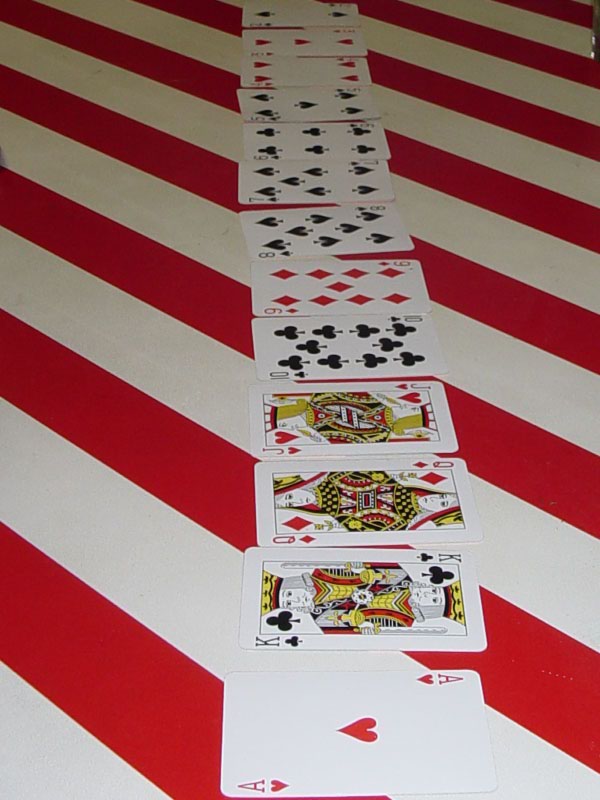The image displays a sequence of playing cards arranged in a neat vertical line from bottom to top. At the very bottom is the Ace of Hearts, followed by the King of Clubs. Above the King is the Queen of Diamonds, then the Jack of Hearts, the 10 of Clubs, the 9 of Diamonds, the 8 of Spades, the 7 of Spades, the 6 of Spades, the 5 of Spades, the 4 of Hearts, the 3 of Hearts, and finally, the 2 of Spades at the top. The cards are placed against a background that features diagonal red and white stripes, running from the top left to the bottom right, with alternating white and red segments enhancing the visual appeal.